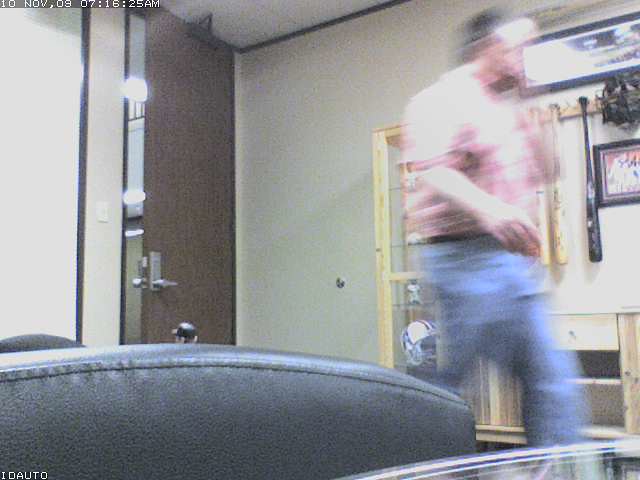The image captures the interior of a personal room, brimming with sports memorabilia. Prominently displayed are several baseball bats hanging from a shelf, alongside a glass cabinet that showcases an American football helmet at the bottom. These items suggest the room is located in North America, likely the USA. A man, wearing blue jeans and a pink polo shirt, is walking past the cabinet. His movement is slightly blurred, indicating the photo was taken quickly, as he strides to the right of the frame.